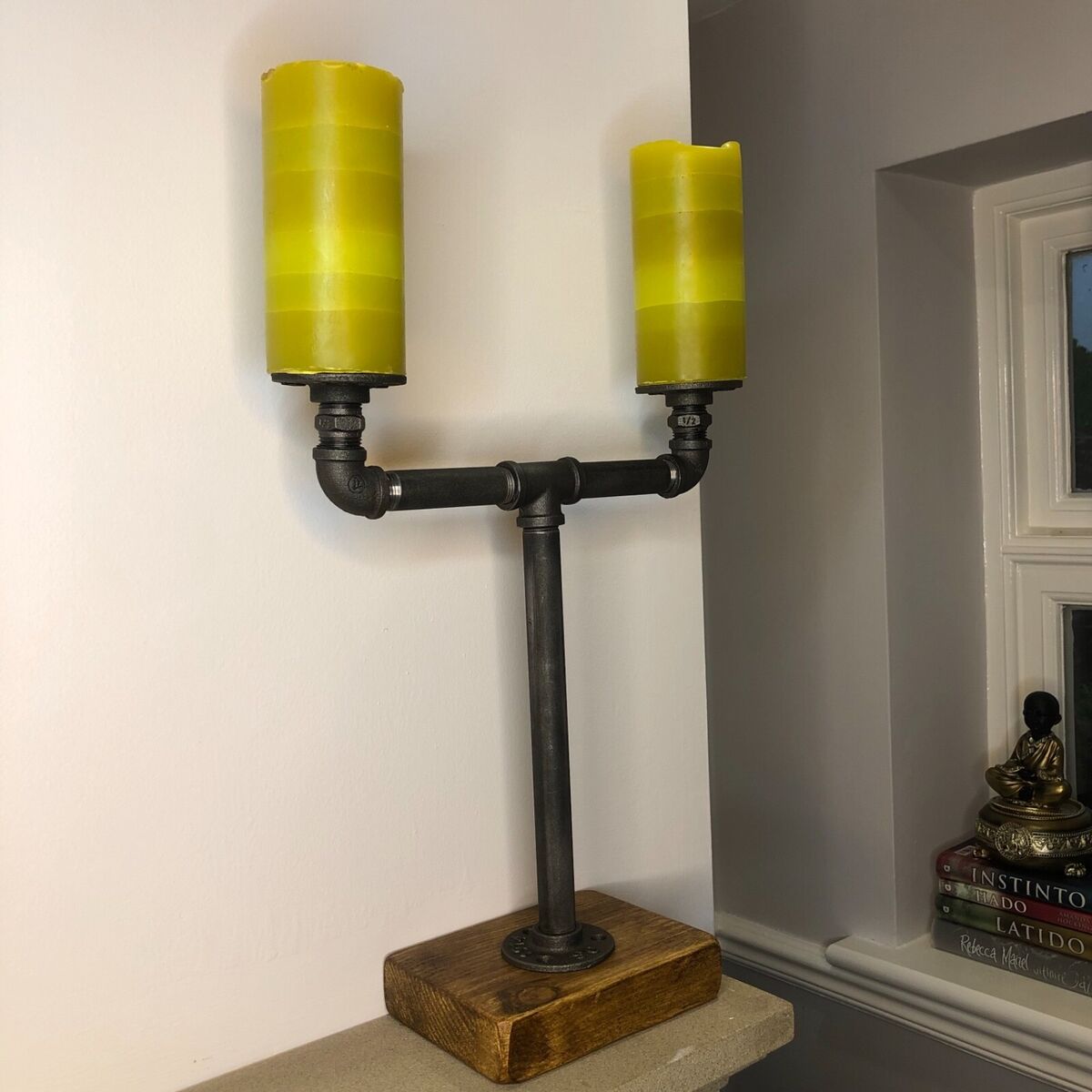The image depicts a steampunk-inspired candelabra with an industrial design, placed on a light brown stone shelf in the hallway of a home. The candelabra features a rectangular wooden base with a dark stain, and a prominent black metal pipe that rises more than a foot before branching into two arms. Each arm supports a circular metal base, upon which rests a large yellow candle adorned with stripes of a darker yellowish-brown color. The candles appear new and match in size and color. In the background, there is a white wall, which appears grayish in the lighting, and a recessed window with white molding. Adjacent to the candelabra, a smaller white shelf holds four stacked books with visible white titles and a small golden Buddha statue resting on top.